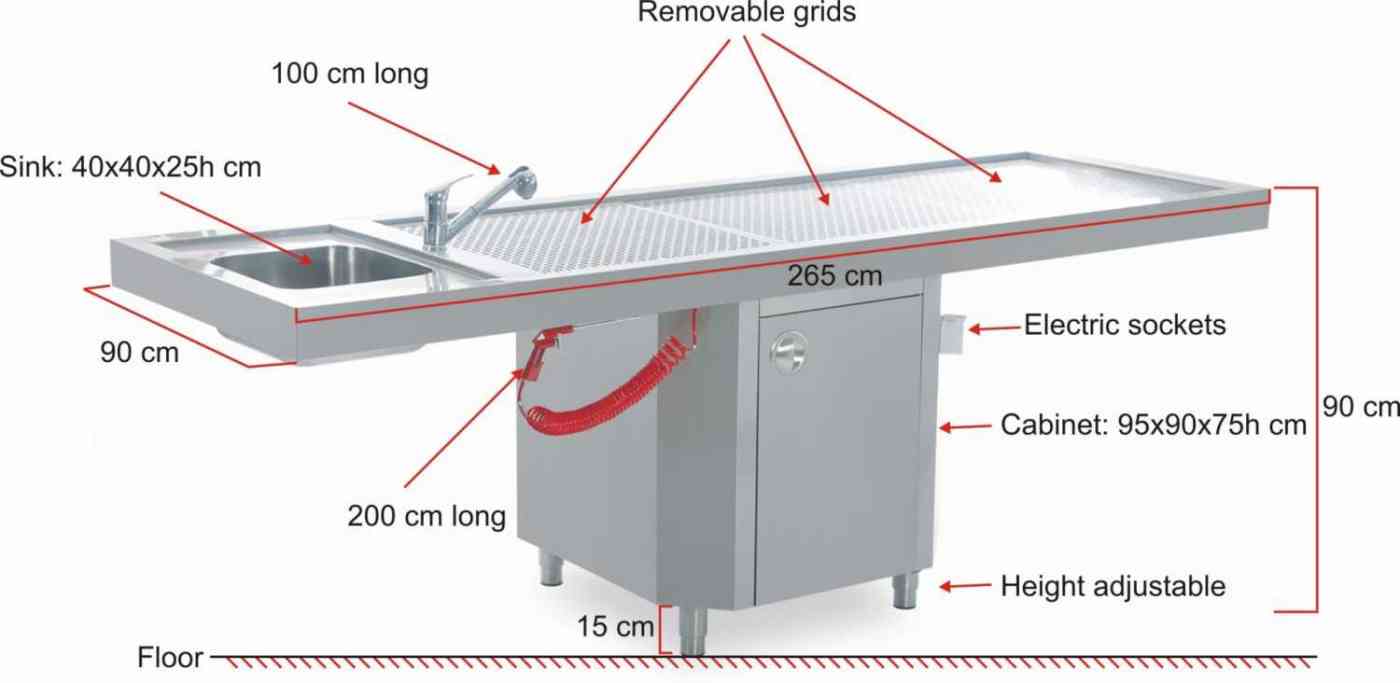This detailed illustration showcases a commercial sink setup, designed for professional use. On the left side of the drawing, the main feature is a sink with specified dimensions of 40 cm in length, 40 cm in width, and a height of 25 cm. Above the sink, there is a faucet rendered in a metallic gray color, accompanied by annotations indicating its length of 100 cm. 

Adjacent to the sink are removable grids, marked by three red arrows, suggesting their functional placement. The entire sink and countertop assembly is situated atop a sleek metal cabinet, also in a cohesive gray tone. The illustration labels the cabinet with dimensions of 95 cm in length, 90 cm in width, and 75 cm in height. Additionally, the height from the top of the removable grids to the floor is specified as 90 cm, with adjustable legs that are 15 cm long, clearly marked in red.

Below and near the cabinet is a sprayer equipped with a red hose, noted to be 200 cm in length. To the right of the illustration, an electric socket is clearly identified, providing a practical detail for electrical connectivity. Words and arrows surround the image, providing clarity for each component and measurement.